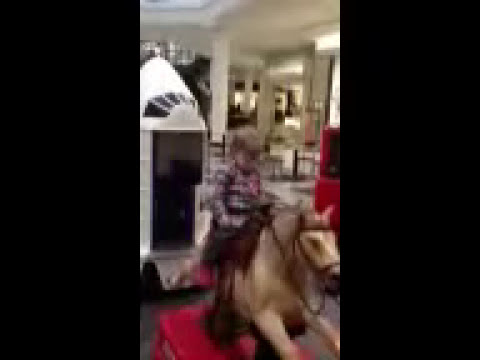A young child, likely a toddler, is sitting on a beige mechanical horse with a red base, situated in what appears to be a mall play area. The child is dressed in a checkered long-sleeve shirt, dark pants, and red shoes. The horse has a dark harness that the child is holding onto. The image, taken with an older camera or phone, is quite pixelated and slightly blurry. In the background, other mall rides can be seen, including a distinctive white space shuttle ride with a black opening. The surroundings include shiny white tiles, white columns, a red booth, and what appear to be retail store fronts, suggesting the typical decor of a shopping mall.